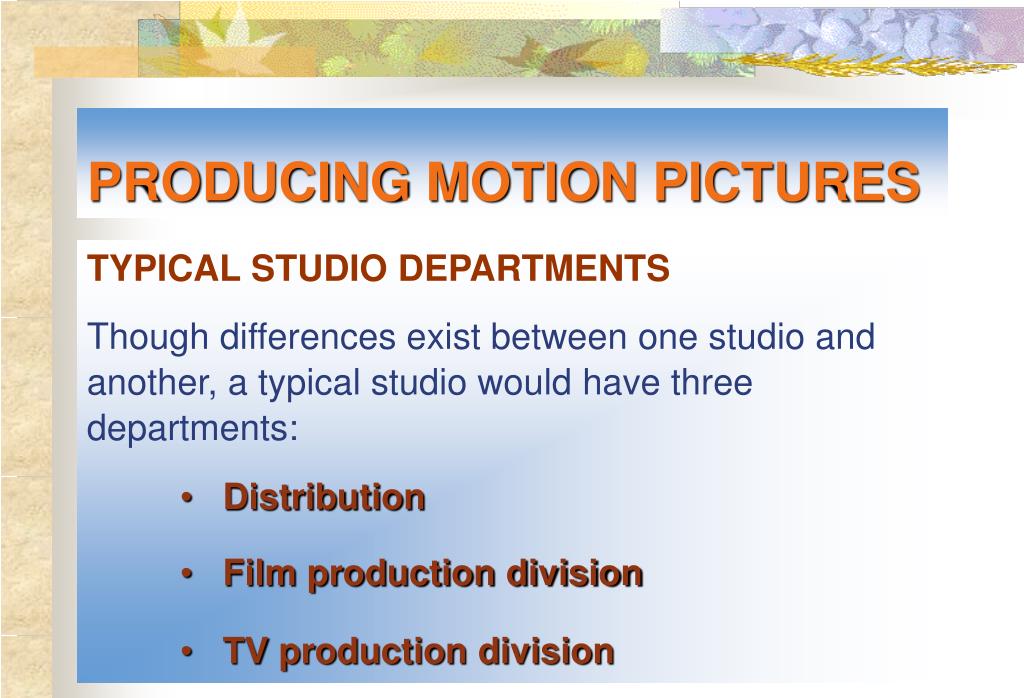The image appears to be a slide from a PowerPoint presentation, framed with a generic floral border that adds a touch of color along the top and left side. The background of the slide transitions smoothly from blue to white back to blue, creating a gradiated effect. Over this backdrop, there is a header in orange text that reads "Producing Motion Pictures." Below this, in red text, is the subtitle "Typical Studio Departments." Further down, a paragraph in blue text explains, "Though differences exist between one studio and another, a typical studio will have three departments." This section is followed by three bullet points—Distribution, Film Production Division, and TV Production Division—listed in red text. Overall, the slide is predominantly focused on textual information rather than imagery, with its content formatted on a neat blue and white background.